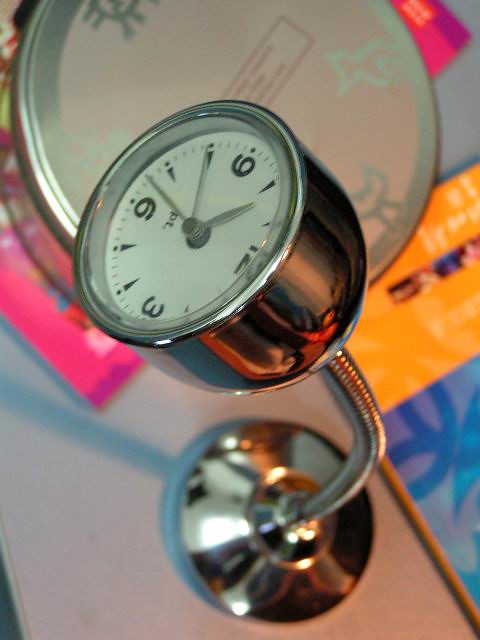This photograph features a sleek, all-metal clock predominantly made of silver. The clock rests on a silver base, which connects to a flexible, bendable neck also in silver. The clock itself has a silver frame, and its face is white with the numerals 12, 3, 6, and 9 prominently displayed; the remaining positions are marked by small triangles. The clock is positioned so that it tilts toward the top left-hand corner of the image, presenting an upside-down view to the observer. In the blurred background, the clock appears to be situated on a desk, accompanied by a stack of books. One book is blue and orange, while another is pink with a metallic tin placed on top of it, adding a splash of color and texture to the scene.